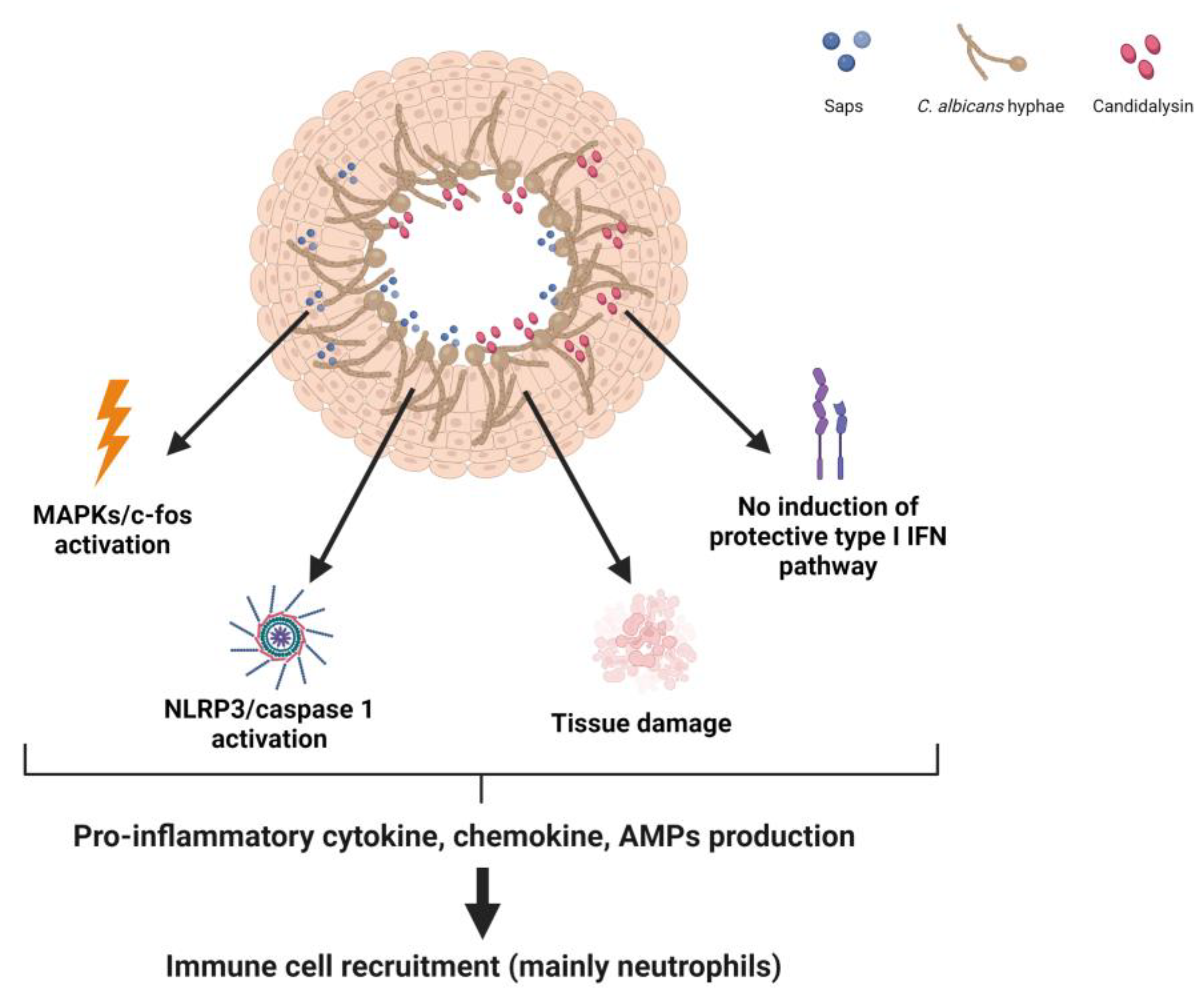The image is a detailed scientific diagram featuring a pale pink, donut-shaped structure on the left side, representing a cellular environment. Surrounding this pink donut are small beige squares with dots inside. Emerging from the center are beige lines resembling twigs, which end in small circles. These represent C. albicans hyphae. Scattered across the donut are small blue and pink circles, identified by the key at the top right; the blue circles are saps, while the pink circles are candied allicin. 

From the bottom half of the donut, four labeled arrows extend outward. The first arrow, marked with an orange thunderbolt, indicates MAPKS/C-FOS activation. The second arrow, symbolized by a blue and pink sun, denotes NLRP3-CASPASE1 activation. A third arrow points to a pink mass that appears as a cluster of small circles, labeled tissue damage. The fourth arrow, featuring shapes like purple and blue mascara wands, describes the lack of induction of the protective type I IFN pathway.

Beneath these arrows, a line leads to text reading pro-inflammatory cytokine, chemokine, and AMP production. Finally, a bold black arrow points to text stating immune cell recruitment, mainly neutrophils, summing up the immune response depicted in the diagram.